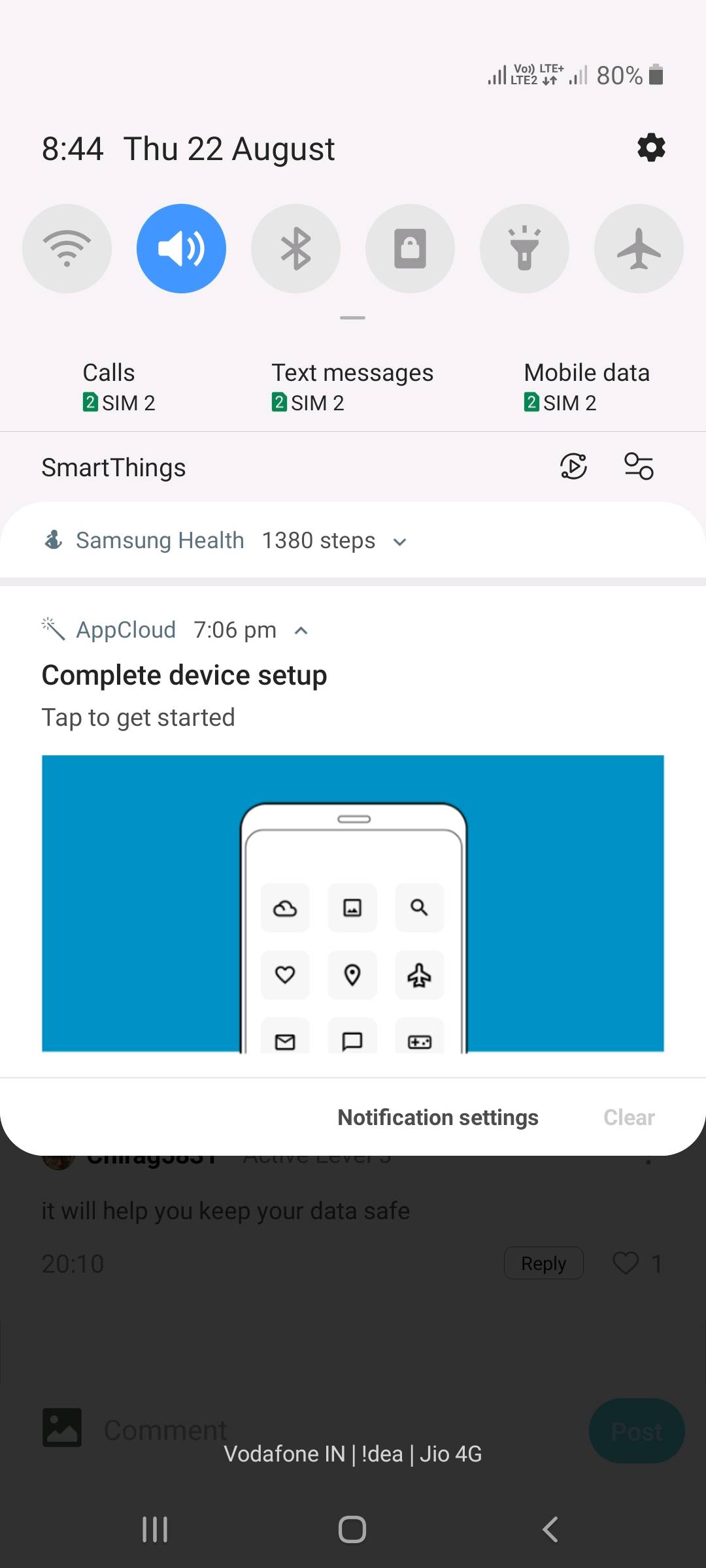The image features a smartphone screen with a light gray background at the top displaying the time "8:44" and the day "THU, 2-2 August" in black text. Below the time, there are six circular icons arranged horizontally. The first icon is a gray Wi-Fi signal icon, the second icon is blue and white with a speaker sound symbol, the third icon is gray with two triangular lines, the fourth icon is a gray lock, the fifth icon is a gray flashlight, and the sixth icon is a gray airplane. Above the airplane icon, there is a black gear symbol next to text in gray that reads "80%."

Below the icons, text indicates "calls SIM 2, text messages SIM 2, mobile data SIM 2" followed by a black horizontal line. The section below this line displays "SmartThings" in black text and "Samsung Help" in white text. Another line of text mentions "1,300 steps" alongside a thin gray horizontal line.

Further down, there is text that reads "App Cloud, 7:06 PM" in smaller black font, followed by a bold black text "Complete device setup" and a red and black prompt stating "Tap to get started." Below this, a blue rectangle is visible. The lower portion of the screen shows a black and white separation line, with "Notification settings" written in black and "Clear" with a capital 'C' in gray just below.

The overall image captures the organization of various notifications and settings icons on the screen, with a detailed layout of both visual and textual elements.